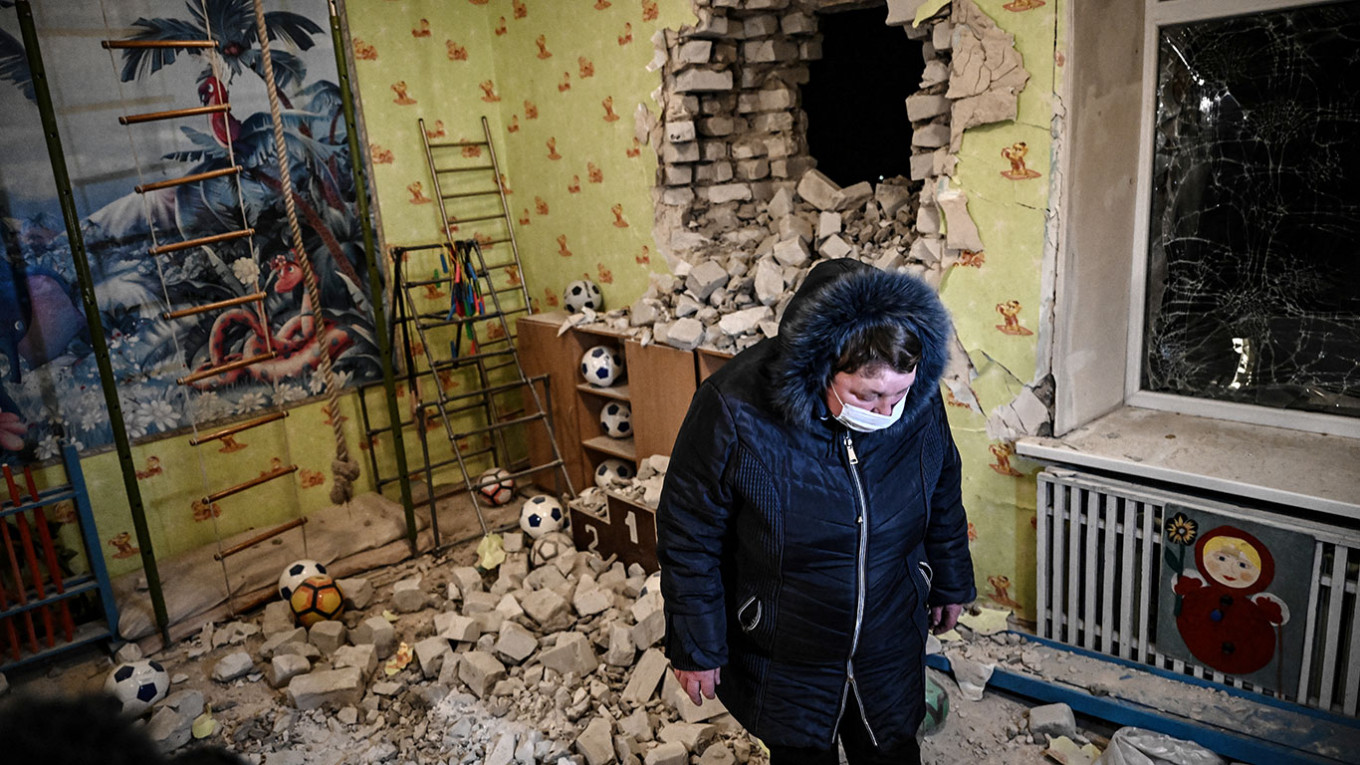The color photograph depicts a woman wearing a blue winter coat with a fur-trimmed hood and a medical face mask. She stands amidst the chaotic interior of what appears to be a children's room, severely damaged by an apparent blast. The thick concrete wall has a gaping hole, with broken bricks and rubble scattered below. To the right of the hole, a window is shattered. Various items typical of a child's room, including multiple soccer balls on the floor and shelves, and a large rope ladder hanging from the ceiling, are visible. The back wall features a large poster displaying a nature scene, juxtaposed against the destruction.